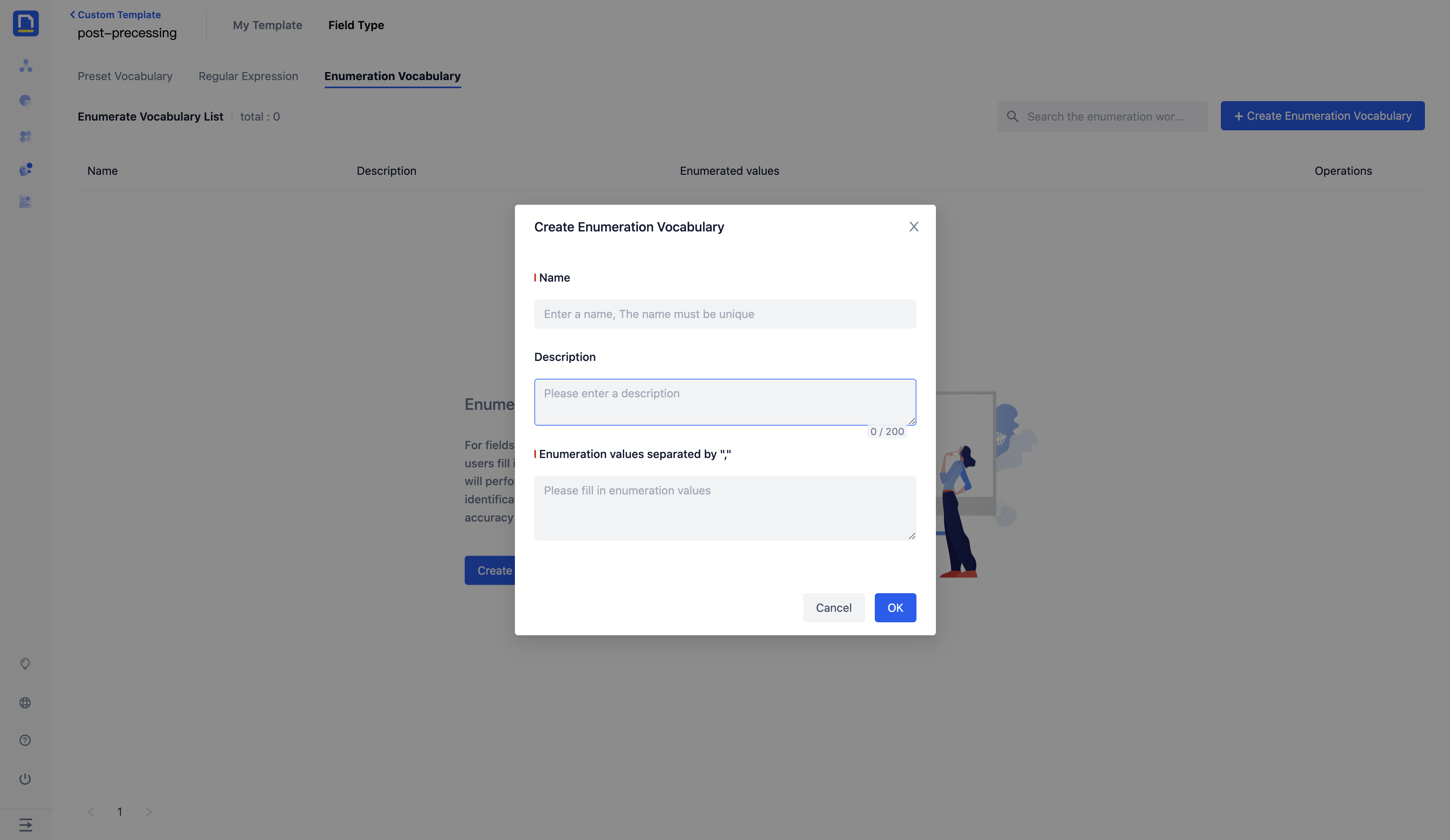The image showcases a website interface featuring a custom template for post-processing. In the upper left corner, there is a label that reads "Preprocessing" followed by "My Template Field Type." This section is overlaid with a semi-transparent gray film. Dominating the center of the screen is a white pop-up modal titled "Create Enumeration Vocabulary."

Within the pop-up, there are several data entry fields. The first field is labeled "Name," with a placeholder text in gray that instructs users to "Enter a name" and notes that "The name must be unique." Below this field is a section captioned "Description," accompanied by a gray text box outlined in blue where users are prompted to "Please enter a description." This text box also indicates that users can input up to 200 characters, with the current character count displayed as "0 of 200 characters can be used" in a darker gray font.

Further down, there is a field labeled "Enumeration values (separated by quotes "")." This section requests users to input enumeration values separated by commas and enclosed in quotes. The gray data entry field for the enumeration values also features a darker gray instructional text and includes the functionality to be resized by dragging the handles at its bottom right corner. Both the "Description" and "Enumeration values" fields offer the flexibility to expand for a more comfortable data entry experience.